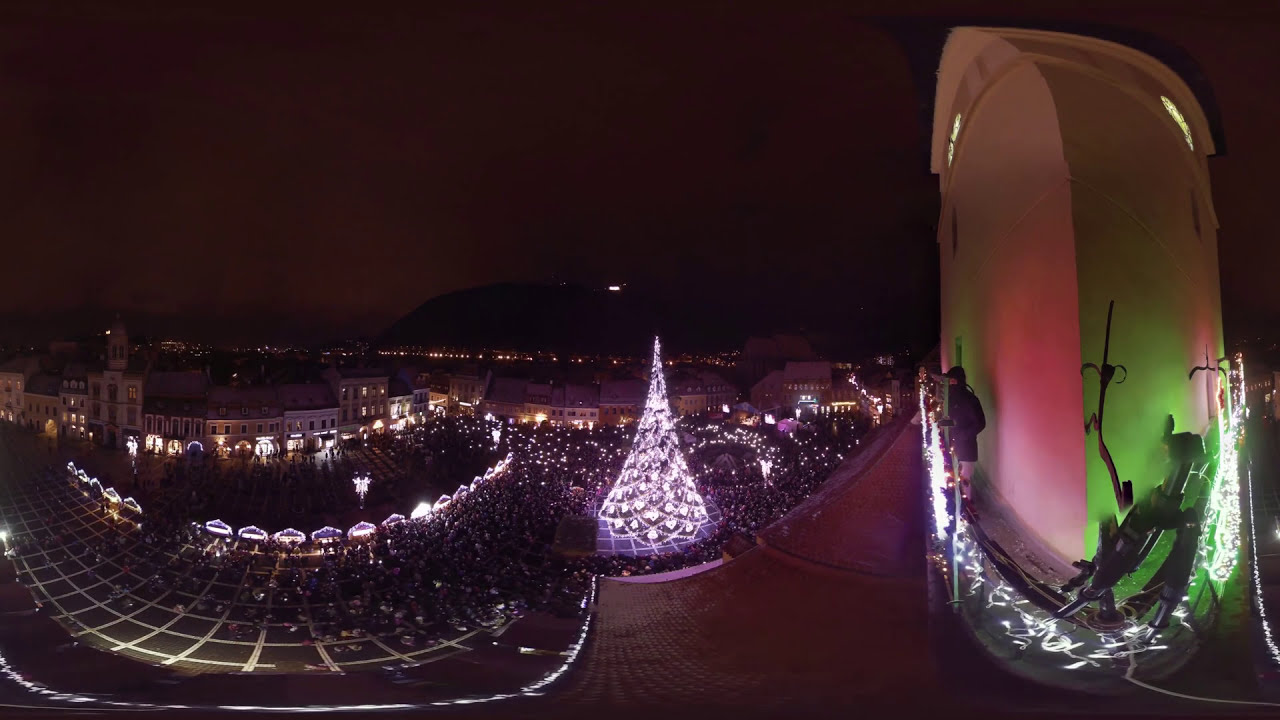The image captures a bustling nighttime Christmas festival scene in a downtown plaza, likely taken with a 360-degree camera, which adds a unique warped perspective. At the center stands a towering, white Christmas tree adorned with intricate white lights, giving the impression of leaves spiraling up to the top. Surrounding the tree, a large crowd of people gathers, perhaps holding candles or other lights, adding to the festive ambiance. On the left side, a series of illuminated booths with triangular, pointy roofs line up, emanating warm holiday cheer. To the right, a large white tower appears distorted at the top due to the camera’s effect, and next to it is a reflective window with pink and green tones, adding an artistic touch. The dark skyline forms a backdrop, emphasizing the brightly lit decorations and the lively crowd below. A person in a black jacket, potentially the photographer, stands on a balcony overlooking the scene.